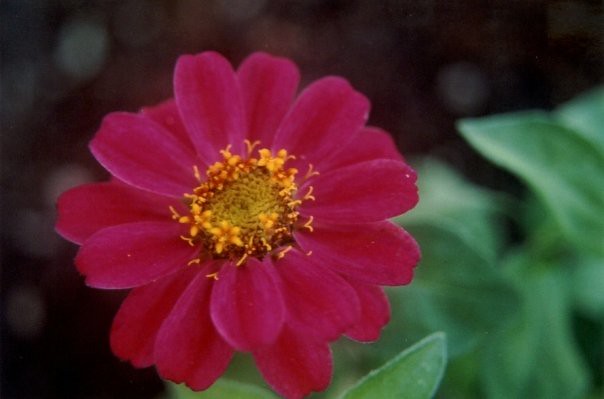This close-up, landscape-oriented color photograph captures the vibrant blossom of a zinnia in stunning detail. The zinnia, positioned slightly to the left and occupying a significant portion of the image, showcases petals that range from a bright reddish hot pink to fuchsia with lighter pink edges. The rosette-like arrangement of its numerous, narrow petals gives it a resemblance to a rose. At the flower’s center, yellow stamen and stigma stand out prominently, with additional small yellow flowers blooming at the edges. The innermost part of the center displays a grainier, dirtier yellow hue. Surrounding the flower, blurred spear-shaped green leaves, similar in appearance to smooth mint leaves, subtly frame the scene. The background fades into a darker, out-of-focus area, indicating a cloudy daylight setting while enhancing the focus on the zinnia's vibrant color and intricate structure.